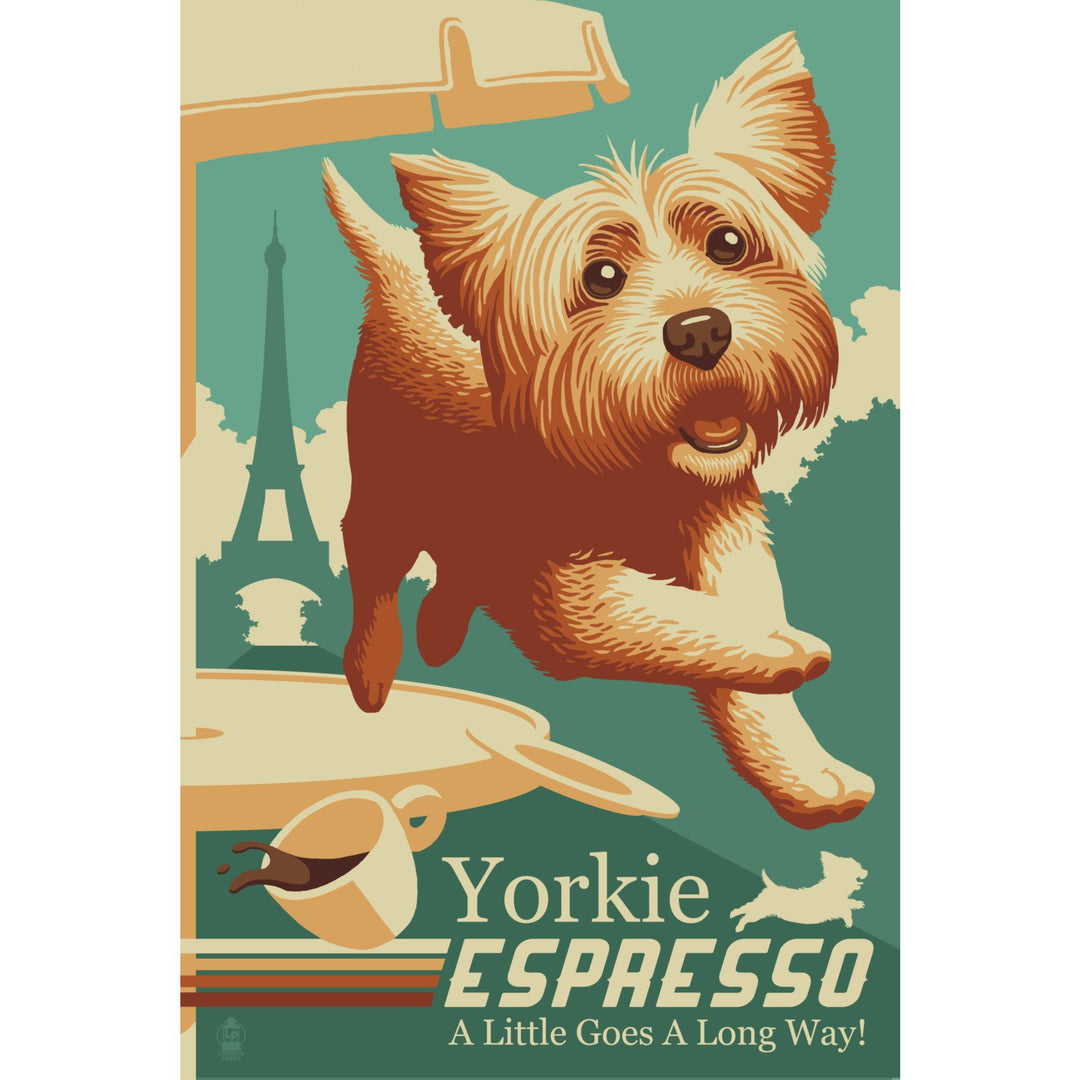This vertically aligned rectangular image, likely a cover for a magazine or book, presents a lively scene featuring a vibrant, animated Yorkie. The background suggests an outdoor café setting with half a table and umbrella visible on the left side. A coffee mug and plate are seen flying off this table, spilling coffee into mid-air, presumably knocked over by the energetic Yorkie. The close-up view showcases the dog’s brown eyes, pointy ears, brown nose, open mouth, and short tail, all contributing to its expression of surprise and dynamism. 

The background gradient combines shades of green, light blue, turquoise, and off-white, and clearly features a faint, outlined silhouette of the Eiffel Tower as well as some trees, hinting at a Parisian backdrop. At the bottom of the image, the text "Yorkie Espresso" is displayed in tan color along with an outlined version of a Yorkie. Below this, the slogan "A little goes a long way!" is vividly printed, encapsulating the playful energy of the scene.